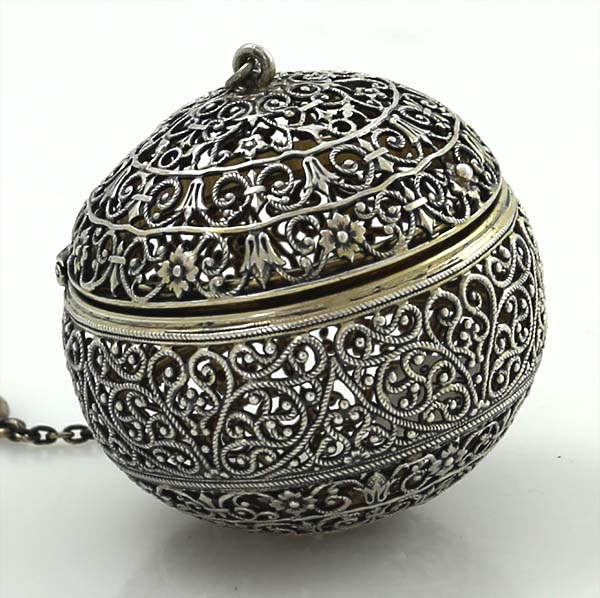The image features an intricate, vintage-style silver tea ball with a detailed filigree scroll design. The tea ball, made of metal and accentuated with black highlights, displays signs of age and use with a slightly worn silver line and hints of gold patina around its edge. It has a hinged lid allowing it to open for placing tea inside and is connected to a small, delicate chain that drapes to the left of the photograph. The tea ball sits on a white table against a white background, emphasizing its ornate design and elegant form. The detailed craftsmanship and decorative elements suggest it may also be mistaken for a Christmas ornament or an incense holder, though it is primarily designed for brewing tea. The square image showcases the delicate balance of its silver and black scroll pattern, making it a visually captivating piece.